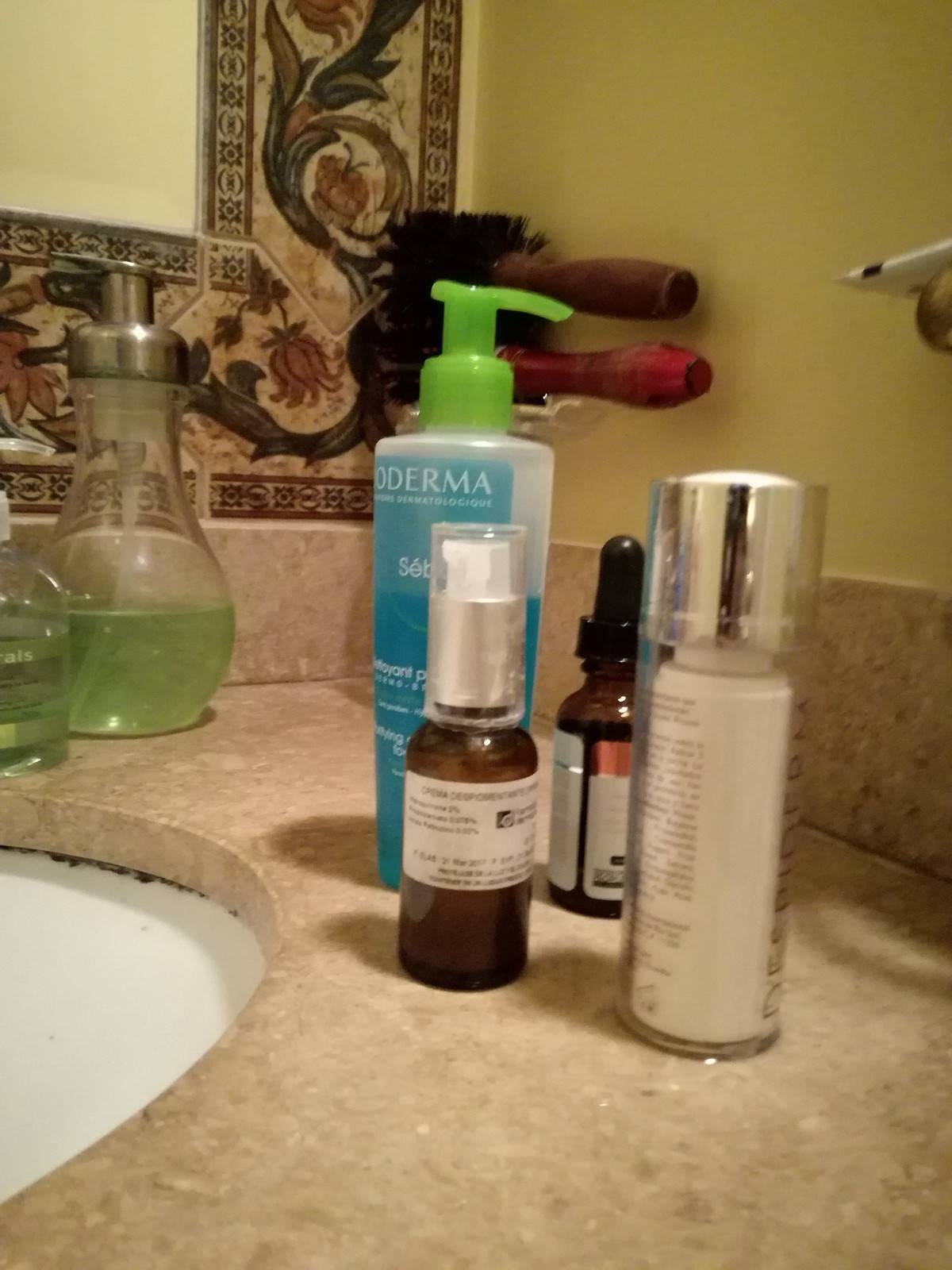The photograph captures a bathroom scene, showcasing the lower left-hand curve of a white, round or oval sink. The surrounding countertop is a speckled tan color. Behind the sink, a mirror with a decorative frame adorned with a dark vine pattern and dull red flowers hangs on the creamy off-white wall. Centrally placed on the countertop are four different product bottles: a tall clear bottle with a blue label and green pump filled with blue liquid, an amber bottle with a white label and white pump, an amber bottle with a black dropper top, and a white bottle with a silver top. Adjacent to the sink on the left are two bottles containing green liquid, likely hand soap. At the top center of the image, two hairbrushes with wooden handles rest on a ledge or shelf.